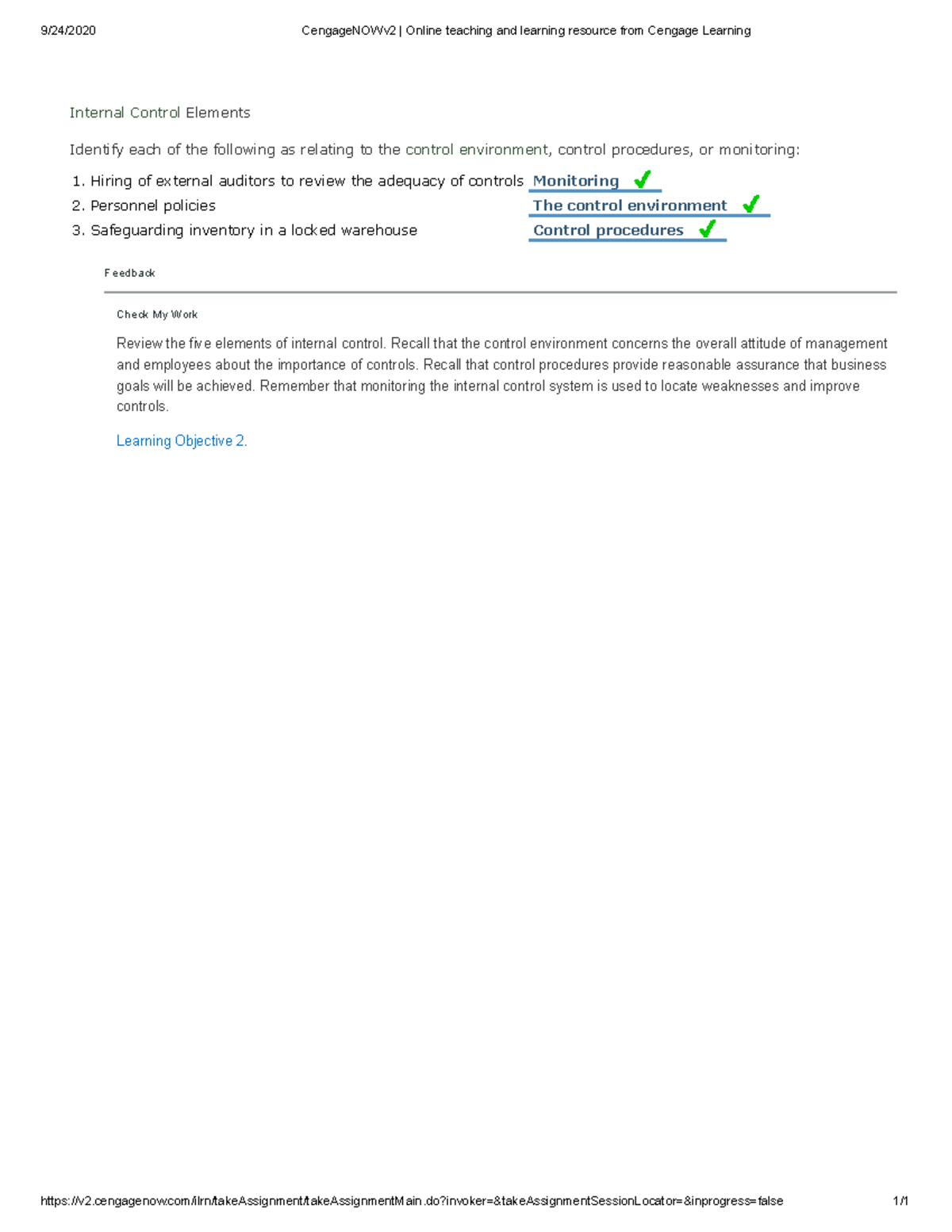Caption: 

The image portrays a digital interface featuring an array of textual information primarily focused on internal control elements in a teaching and learning resource. At the top left, the date is prominently displayed: September 24, 2020. On the top right, there are labels and text including "CengageNow," "V2," and "online teaching and learning resource from CengageLearn." The detailed content revolves around identifying various aspects of internal control, divided into categories such as the control environment, control procedures, and monitoring. The numbered list mentions specific actions—hiring external editors to review the adequacy of controls, implementing personnel policies, and safeguarding inventory in a locked warehouse. The interface also features interactive elements like 'Feedback,' 'Check My Work,' and a detailed review of the five elements of internal control. The explanatory notes underscore the importance of the control environment in shaping management and employees' attitudes toward controls, the role of control procedures in ensuring business goals are met, and the necessity of monitoring to identify and rectify weaknesses within the system.